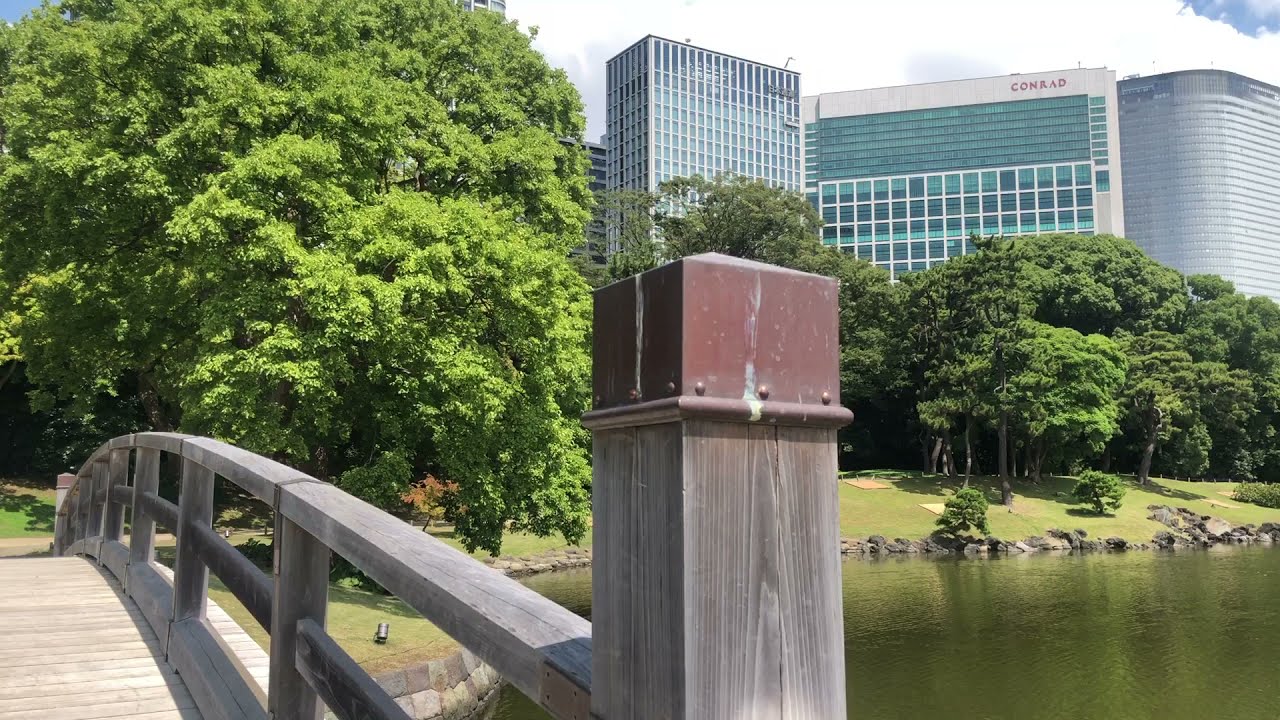A stunning photograph captures a tranquil park with a body of water, appearing to be either a pond or a lake, in the foreground. This green and murky water body, located in the bottom right corner of the image, reflects the lush greenery of the surrounding landscape. Encircling the water is a stone boundary comprised of dark and light gray as well as white rocks. A well-maintained grassy area with scattered bushes and a sloping lawn delineates the edges of the water. Prominently featured in the bottom left is a wooden arched bridge with metal coverings on top of its posts, painted a reddish-bronze color, providing a rustic charm to the scene. A large, vibrant green tree stands at one end of the bridge, while a rich variety of tall trees, smaller trees, and dense bushes populate the background, painting a scene of abundant greenery.

Behind this verdant oasis, a modern office park rises, comprising several sleek skyscrapers, mostly constructed with glass windows in shades of blue, turquoise, and gray. Dominating the skyline are six impressive buildings, among which the middle one bears the text "CONRAD" in bold red letters, suggesting it might be a hotel or another prominent establishment. The architecture is diverse, with the "CONRAD" building being notably wider than it is tall, flanked by a rectangular building to the left and an arched structure to the right. The blue sky above, dotted with white clouds, frames the entire vista, creating a serene yet dynamic cityscape.